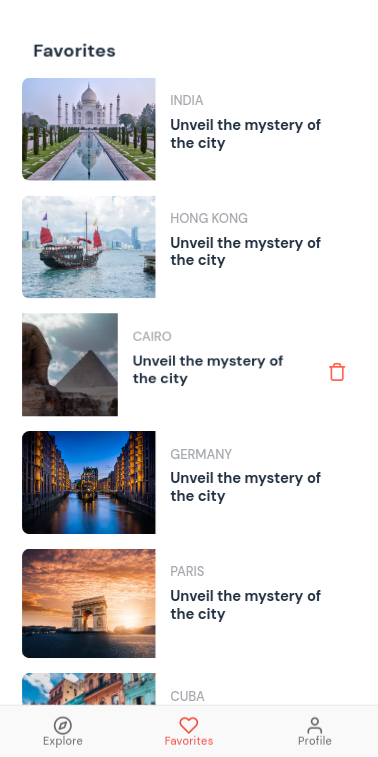This image features a low-resolution, pixelated depiction of selected travel destinations under the heading "Favorites" written in black text on the top left corner against a white background. The blurred and fuzzy quality of the image does not detract from the intention to showcase six different locations, each accompanied by a tagline "Unveil the mystery of the city."

1. **India**: At the top, there is a depiction of a white temple standing majestically by a serene stream. The setting invites viewers to explore the historical and cultural richness of India.
   
2. **Hong Kong**: Below India, Hong Kong is illustrated with an image of a boat floating on a vast body of water, set against a cloudy sky. The scene evokes the vibrant contrast of nature and urban life in this bustling city.

3. **Cairo**: The third highlighted location is Cairo, which features a prominent pyramid on the left side, symbolizing the ancient allure and historical depth of Egypt’s capital city.

Each entry invites viewers to "unveil the mystery of the city," suggesting an exploration of the unique and intriguing aspects of these destinations.